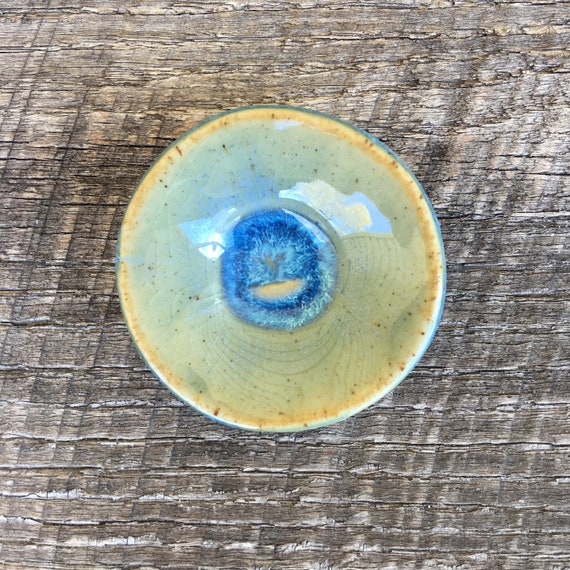The photograph captures a round dish set against a backdrop of gray, weathered wood, showcasing intricate cracks and prominent grain patterns symbolizing its sun-worn history. The dish itself, viewed directly from above, reveals a light yellow interior speckled with subtle variations. Surrounding the rim is a faintly darker yellow hue, accented with hints of blue. The most striking feature is the center of the dish, where a bright blue, eye-like swirl design commands attention, resembling the iris of an eye. This glossy, visually captivating dish stands out as the solitary object on the roughly textured wooden surface, creating a compelling contrast within the image.